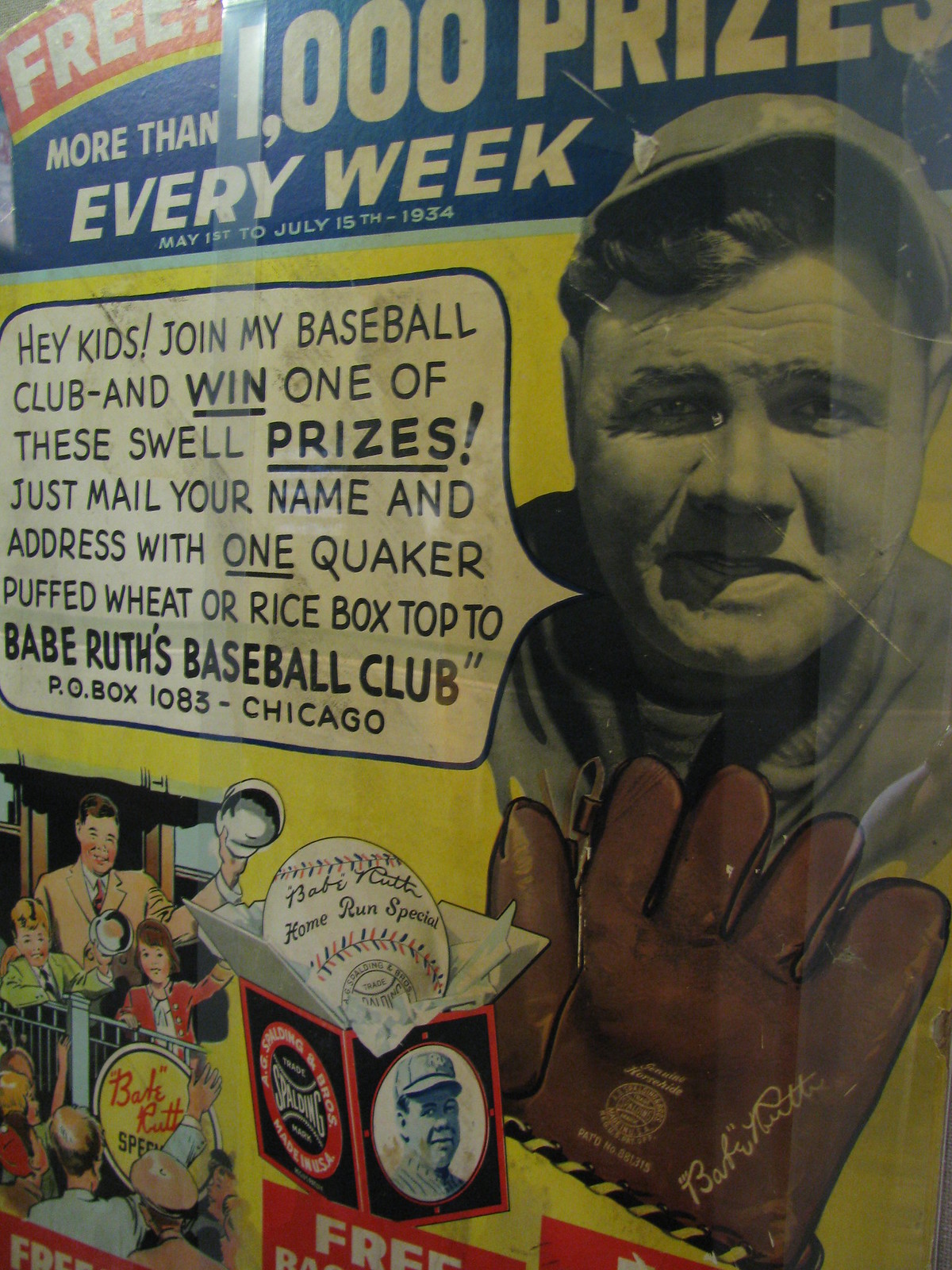The image depicts a close-up of an old advertisement poster from 1934, comprised of multiple pieces taped together to form a larger, cohesive illustration. Dominating the poster are bold white letters on a blue background proclaiming, "Free more than 1,000 prizes every week, May 1st to July 15th, 1934," emphasizing the antiquity and the promotional nature of the poster. Central to the image is a grayscale photograph of Babe Ruth, adorned with a text bubble that reads, "Hey kids, join my baseball club and win one of these swell prizes. Just mail your name and address with one Quaker puffed wheat or rice box top to Babe Ruth's Baseball Club, P.O. Box 1083, Chicago."

Below this section are various smaller illustrations and promotional artworks. To the left, a cartoon depiction features a man and two children enthusiastically waving their hats among a crowd, likely celebrating a baseball scene. Adjacent to this, there's a drawing of Babe Ruth's signed baseball glove and a "Home Run Special" baseball box featuring his face and autograph. The poster, set against a vibrant yellow background, is rich with vintage baseball iconography, encapsulating the spirited marketing style of the early 20th century.